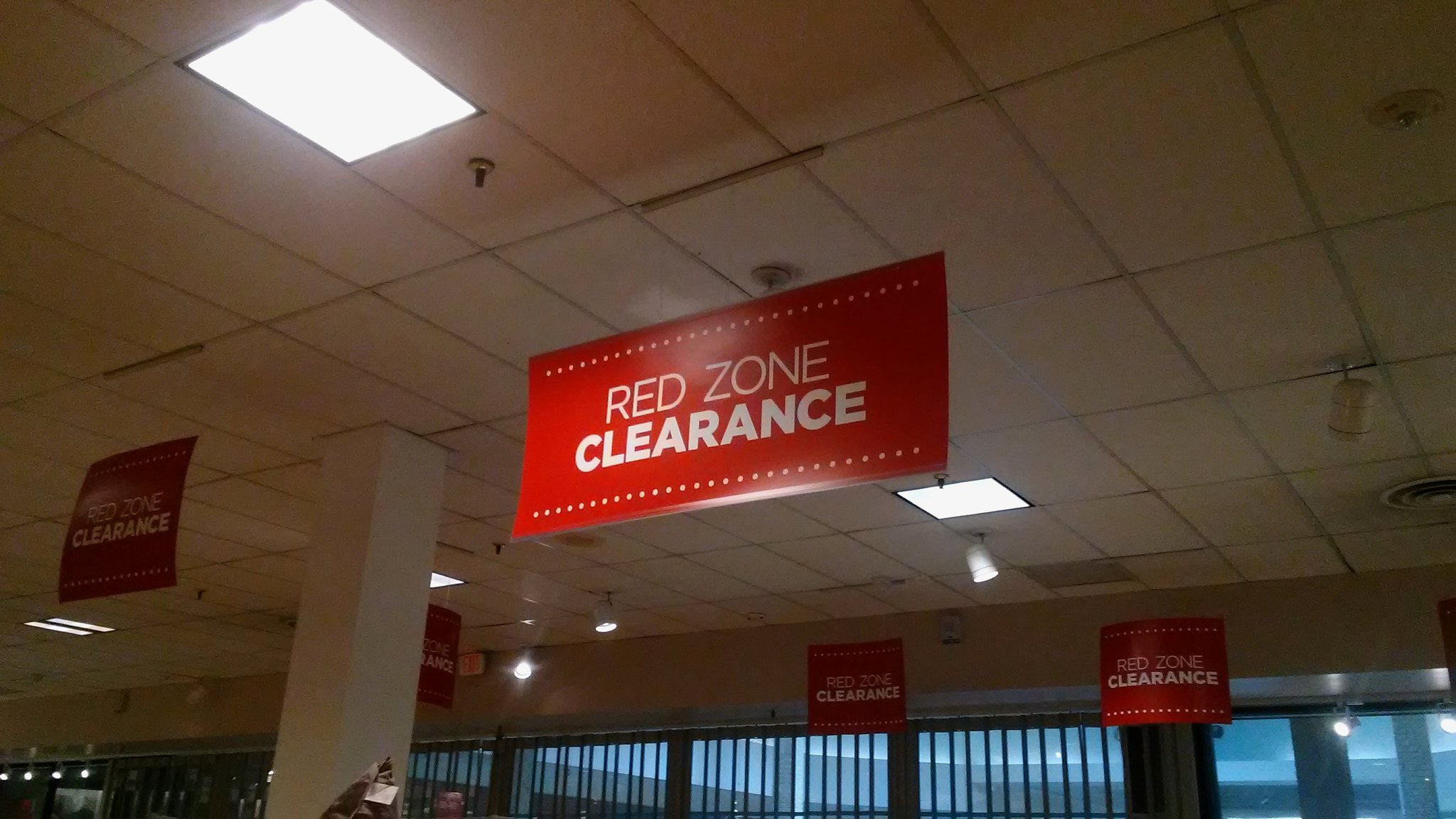This image depicts the interior of a department store, specifically focusing on its ceiling and the prominent "Red Zone Clearance" sale signs. The white-tiled ceiling, slightly worn, features rectangular panels and embedded white lighting that almost occupies half a panel, with one distinct fixture positioned in the top-right corner. Fire sprinklers, silver in color, are also visible amidst the ceiling panels. White columns descend from the ceiling, with one noticeable column about a quarter from the right side of the image. Slatted blinds cover the windows, which are located to the left, nearly three-quarters into the frame, hinting at a dreary outside atmosphere and possibly indicating the store is closed or preparing to open.

Dominating the scene are several red rectangular signs with white dots or stars adorning the top and bottom, prominently displaying "Red Zone Clearance" in bold white lettering, with "clearance" particularly emphasized. One sign hangs about a panel and a half below the light in the top-right corner, while more identical signs are visible in the background near the windows and beyond the columns, suggesting a widespread clearance sale throughout the store. A faint figure of a person, possibly a store employee, is discernible at the bottom center, adding a subtle human element amidst the predominantly structural and signage-focused composition.